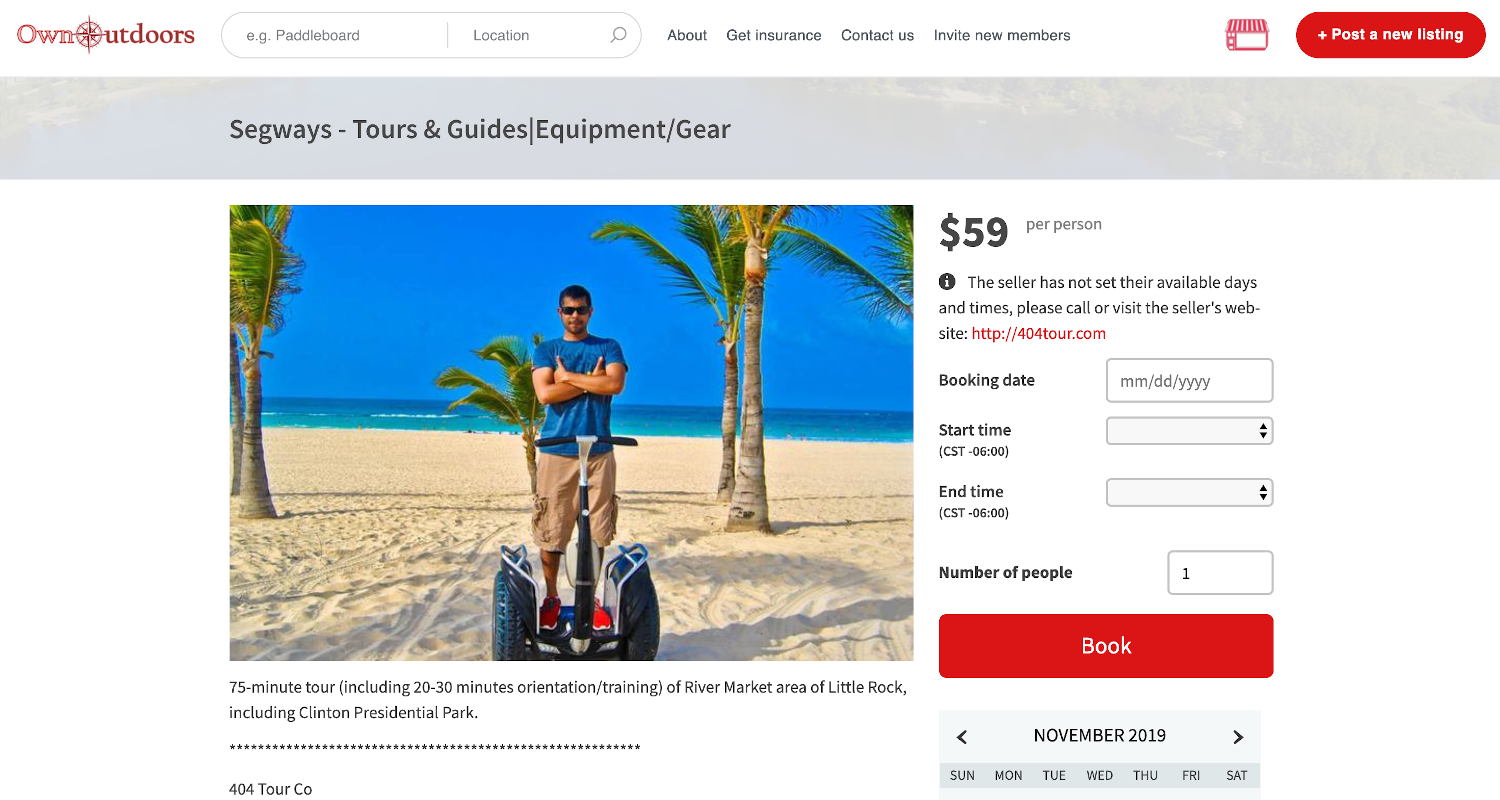The horizontally rectangular image depicts a detailed online retail listing on the Own Outdoors platform.

At the top left, the Own Outdoors logo is prominently featured, adjacent to a search field that currently reads "EG Paddleboard." This search field is designed to help users find specific gear. To the right of the search bar are several navigation links—About, Get Insurance, Contact Us, and Invite New Members. Dominating the upper right corner is a bold red button labeled "Post a New Listing."

Directly below this navigation area is a light gray horizontal banner. In black lettering within this banner, various categories are listed: Segways, Tours and Guides, Equipment, Gear.

The main content of the listing showcases an image of a gentleman on a Segway, positioned on a beach lined with palm trees, against the backdrop of serene water. The tour being offered is a 75-minute adventure including a 20 to 30-minute orientation training, designed to explore the River Market area of Little Rock, which includes the Clinton Presidential Park.

To the right of the image, the price is clearly marked at $59 per person. Notably, the seller has not specified available days and times for the tour. Instead, potential customers are directed to call or visit the seller's website for more information.

Below this information, there are fields available for booking: including options to select the date, start time, end time, and number of people. A prominent red “Book” button with white text invites users to finalize their reservation.

At the bottom of the frame, a small calendar for November 2019 is displayed, with navigational arrows allowing users to browse through different months and years for scheduling.